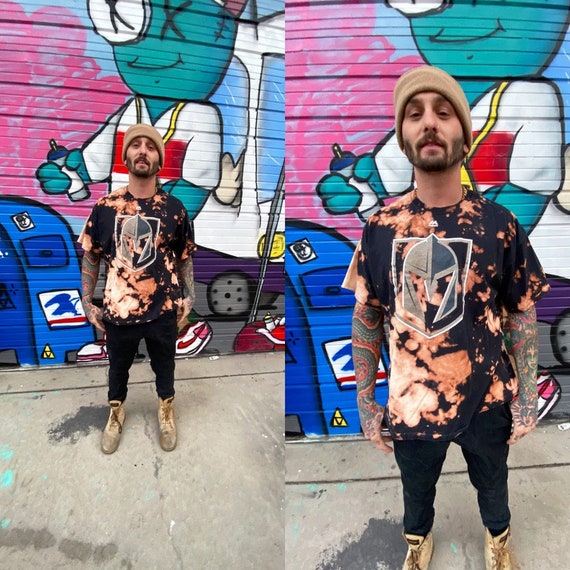This is a two-panel photograph featuring a man standing on a concrete sidewalk in front of a graffiti-covered wall. The image on the left is taken from a slightly further distance, while the one on the right is a close-up of the man. He is wearing black pants and beige lace-up shoes, suitable for urban wear. His shirt is a black and beige bleached tie-dye with a Raiders logo in the center, and he sports a brown knit cap. His arms are covered in colorful tattoos, featuring a mixture of patterns and images, including a woman's face and rainbow-like colors. His facial hair consists of a closely-cropped beard and a black mustache.

The graffiti background is vibrant and intricate, depicting a blue mail drop-box with a blue eagle label and a large blue monster. The monster has a single monocle eye, X-shaped eyes, and appears to be holding a spray can, dressed in a white shirt with red stripes and blue sports shoes, standing in front of a white truck. The concrete ground and the narrow setting suggest an alleyway or an area near a commercial structure.